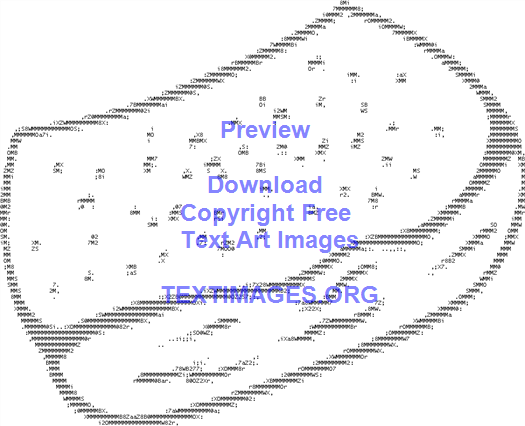The image appears to be a black and white, grayscale clip art of an ambiguous, rectangular-shaped object with a three-dimensional aspect, possibly resembling a sponge, a piece of bread, or a basket. The object has dots on the top and horizontal squiggly lines on the sides, with the left side curving inward. The entire image is outlined in black. Across the image, there is blue text, center-justified, that reads: "preview," followed by "download," "copyright free," "text art images," and "textimages.org." The template-like image seems to serve as an example of digital art available from textimages.org, with the overlay text indicating it is a preview meant for downloading copyright-free text art images.